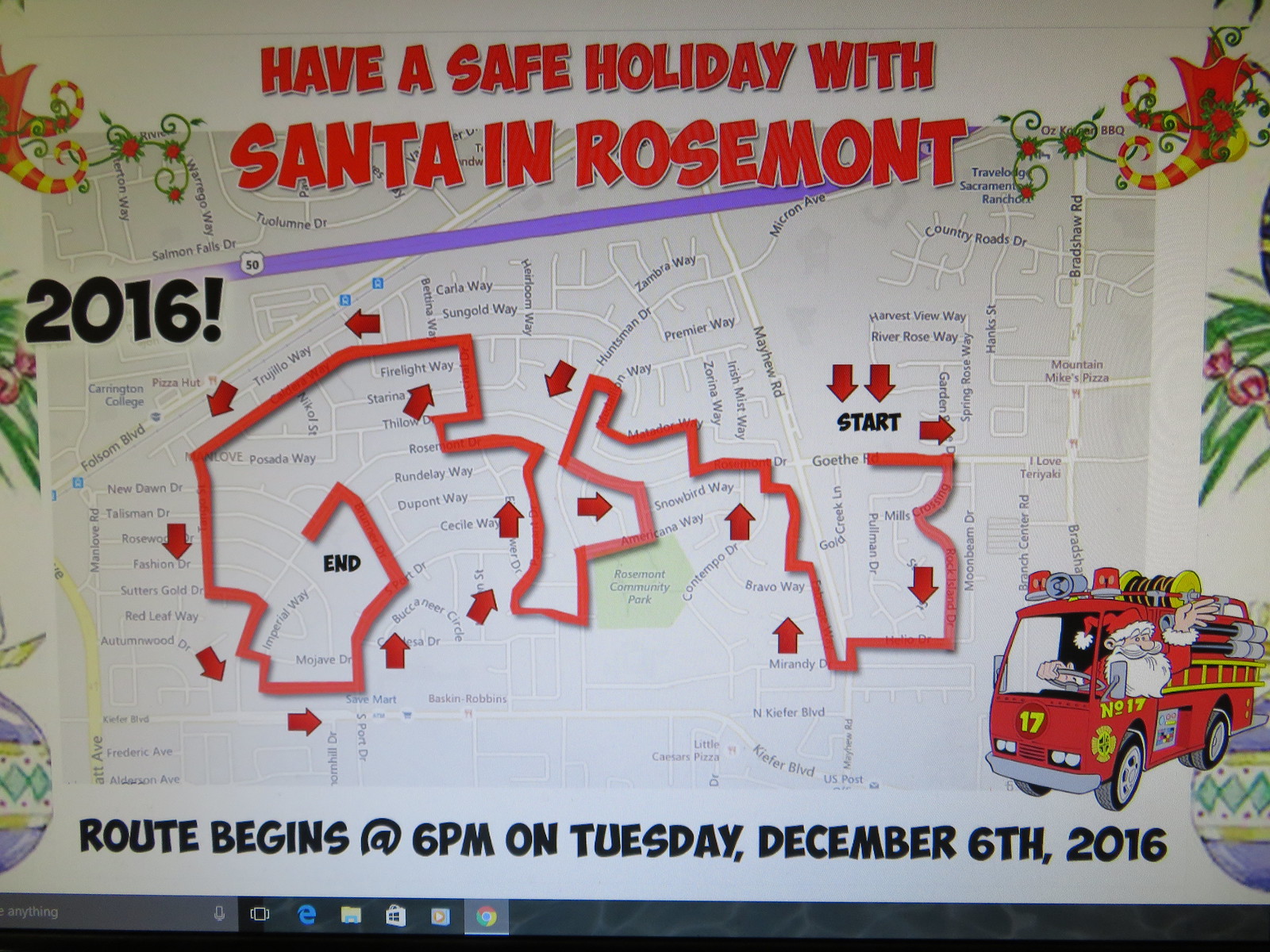A vibrant photo captures a computer screen displaying an online map of Rosemont with a highlighted route starting from point A to point B, marked by directional arrows through a residential area. Topped by large red text that reads, "Have a safe holiday with Santa in Rosemont," the map prominently indicates a festive route charted for a fire truck carrying Santa Claus. The cheerful message is accentuated by Christmas-themed decorations, including jester boots, ornaments, and berries surrounding the map. Noteworthy details include the date "2016" at the top left corner and a playful illustration of Santa waving from a fire truck at the bottom right. The fire truck, distinctly marked with the number 17, is adorned with lights, a yellow ladder, and hoses. The map, viewed within an internet browser, features black text at the bottom announcing, "Route begins at 6 PM on Tuesday, December 6, 2016," ensuring everyone knows when to join in the holiday excitement.